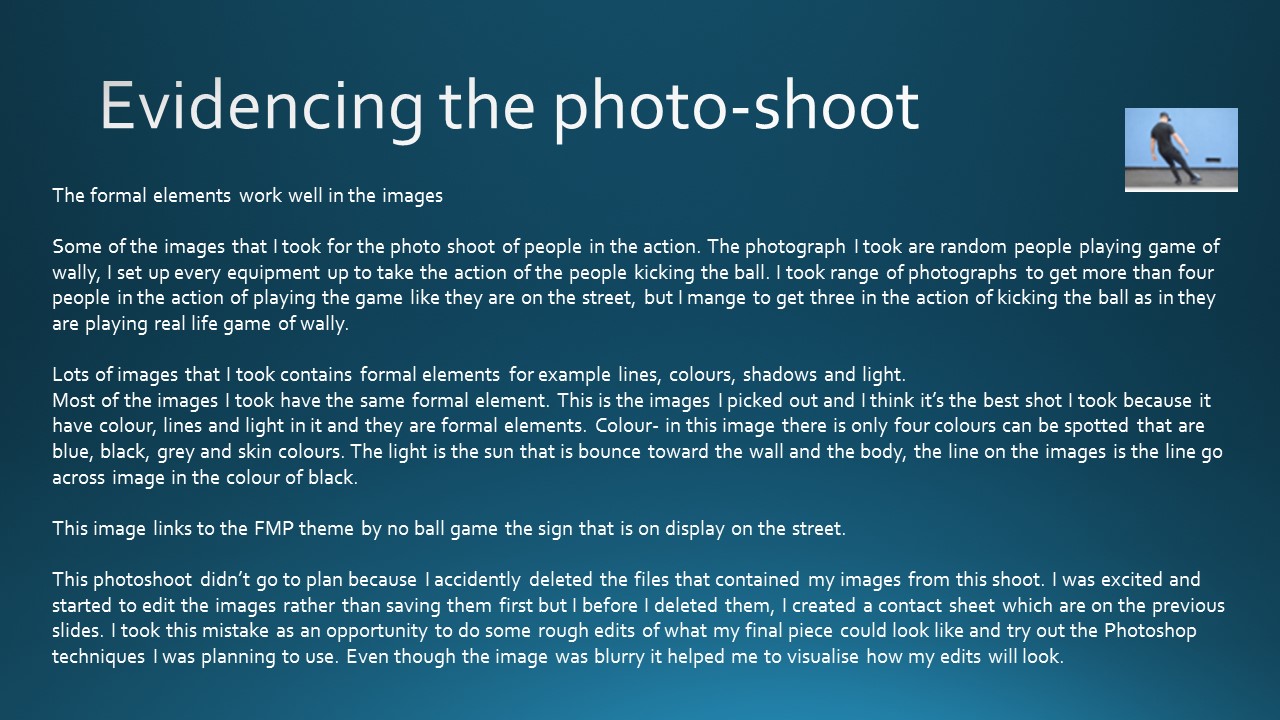The image features a blue gradient background, transitioning from a darker shade at the top to a lighter one at the bottom. On the right-hand corner, there's a small photograph depicting a person dressed in black, leaning backward, possibly while skating up a ramp or performing a dance move. The text on the image primarily describes a photoshoot, detailing the process and experience of capturing people in action.

At the very top, in large white text, the phrase "Evidencing the Photoshoot" stands out. Below this, it reads, "The formal elements work well in the images." The subsequent paragraphs discuss the photographer's effort to capture spontaneous moments of people playing a game referred to as "WALL-E." The photographer meticulously set up the equipment to document individuals kicking a ball, aiming to capture dynamic, street-like scenes. Although they aimed to feature more than four participants, the final images prominently showcase three people engaged in the game. Additional paragraphs provide further insights into the photographer's approach and techniques during this photoshoot.